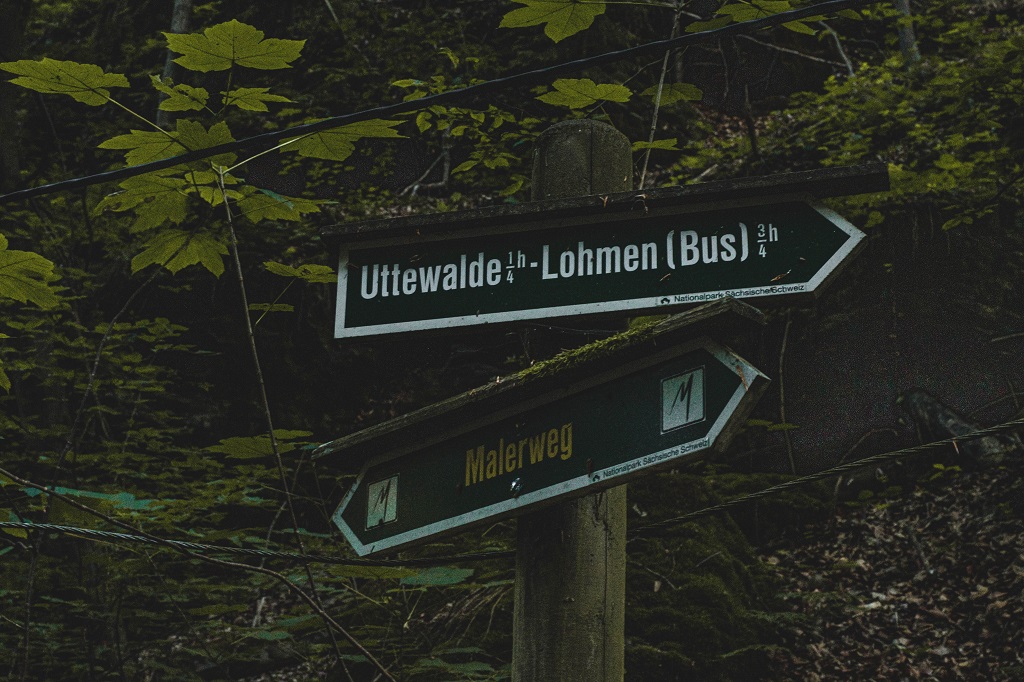The photograph, taken in landscape orientation, features a dense, shadowy forest in the background, filled with leaves, moss-covered rocks, and foliage. The main focus in the foreground is a thick, round wooden post with two weather-protected signs attached to it. Above the signs, wooden planks are fixed, possibly to shield the signs from the elements. The top sign is black with a white border and text; it has an arrow pointing to the right and reads "Uhtewald 1/4 H - Luhmann (Bus) 3/4 H." The bottom sign is also black with a white border and points in both directions. It has yellow lettering that spells "Malerweg," and each side of the text is flanked by a white box containing a black "M." Black cable wires are visible above, but not attached to, the post, extending over and behind it. The overall scene is dimly lit, casting deep shadows across the area and enhancing the natural, untouched atmosphere of the woods.